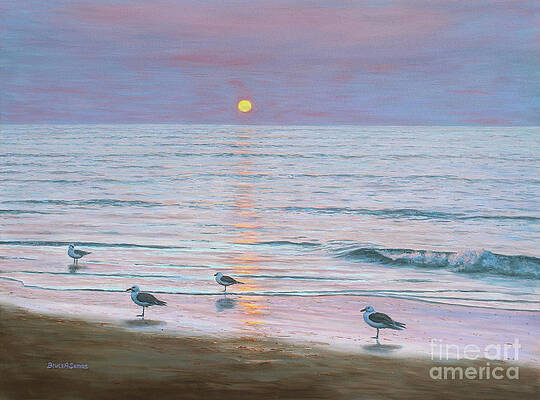The image is a vibrant, almost surreal painting of a sunset over a serene beach, showcasing vivid and slightly unrealistic colors. In the foreground, the shoreline is depicted with brown-colored sand, and gentle, shallow waves crash softly onto the shore, capped with white foam. Four seagulls, with white fronts, yellow beaks, and black-tipped wings and tails, are leisurely perched where the sand meets the shallow water, blending into the tranquil scene. The expansive blue ocean, stretching towards the horizon, is adorned with subtle wave patterns and reflects a touch of purple hue. As your eyes move upward, the horizon meets an enchanting sunset featuring a bright yellow sun. The sunset casts a golden shimmer onto the water, creating a beautiful interplay of light. Above, the sky exhibits a gradient of purplish-blue tones, contrasted by pink-tinged clouds. The painting contains an artist's signature on the lower left, partially readable with the first letter appearing to be a 'D', and a printed mark on the lower right that reads "Fine Art America".